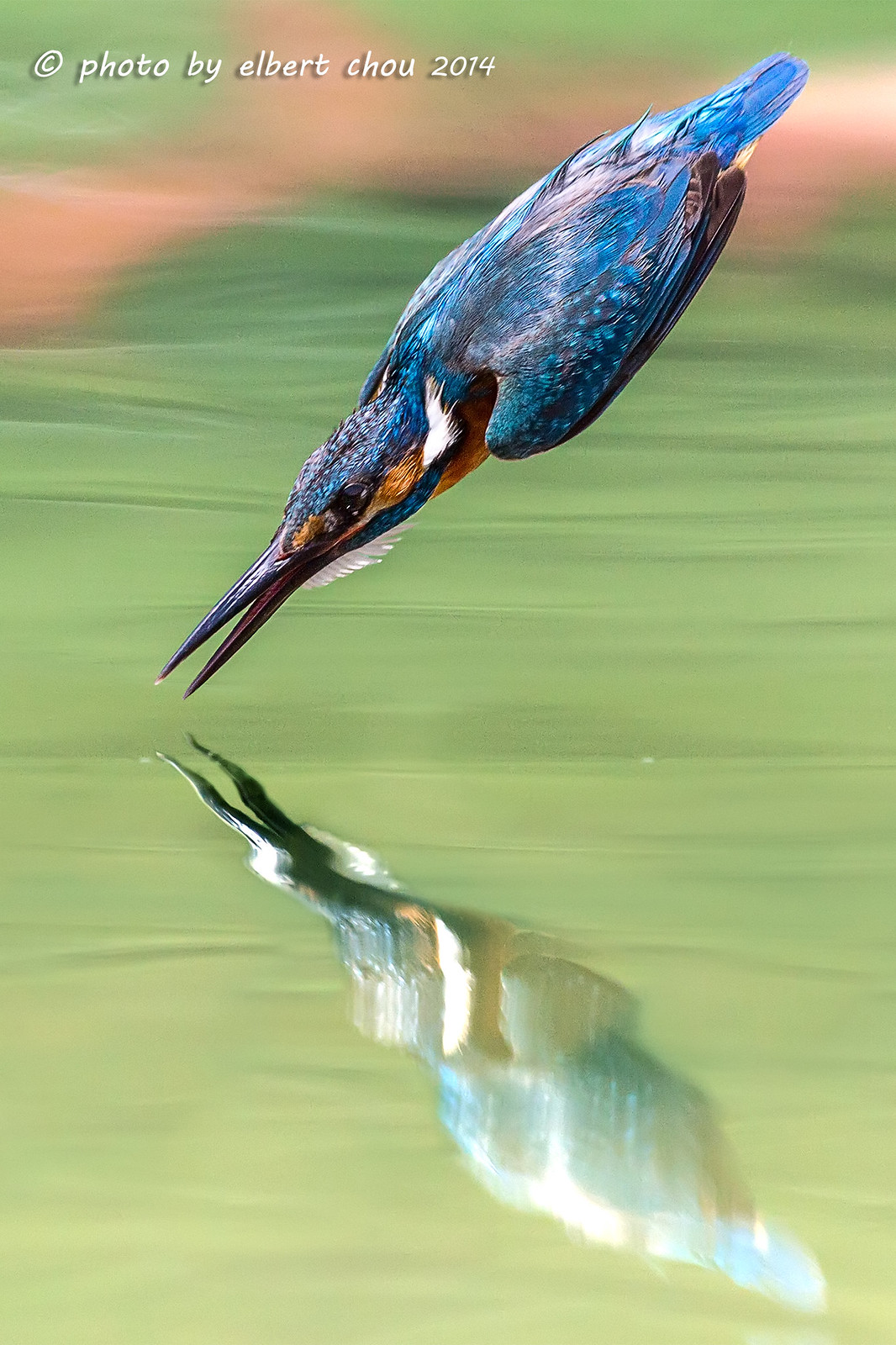This stunning wildlife photograph, captured by Albert Chou (C-H-O-U) in 2014, features a brilliantly blue bird with vibrant orange accents under its eyes and around its beak. The bird, reminiscent of a woodpecker, is captured mid-dive, just about to plunge into green, seaweed-colored water in search of prey, presumably a fish. The bird’s aerodynamic shape is accentuated by its sleek, pointed beak and tightly tucked wings, giving it a streamlined, fierce appearance as it descends rapidly. The photograph is composed such that the bird’s tail feathers are in the upper right corner while its beak points slightly left of center, creating a dramatic diagonal line across the frame. The water below is calm, providing a perfect mirror image of the bird, doubling the visual impact of its vibrant, blue and orange plumage against the green backdrop. The sunny, warm atmosphere of the scene is enhanced by the yellowish tones reflected off the water. The upper left corner of the photograph bears the copyright symbol and the inscription "Photo by Albert Chou, 2014," lending a professional and timeless quality to this exceptional nature shot.